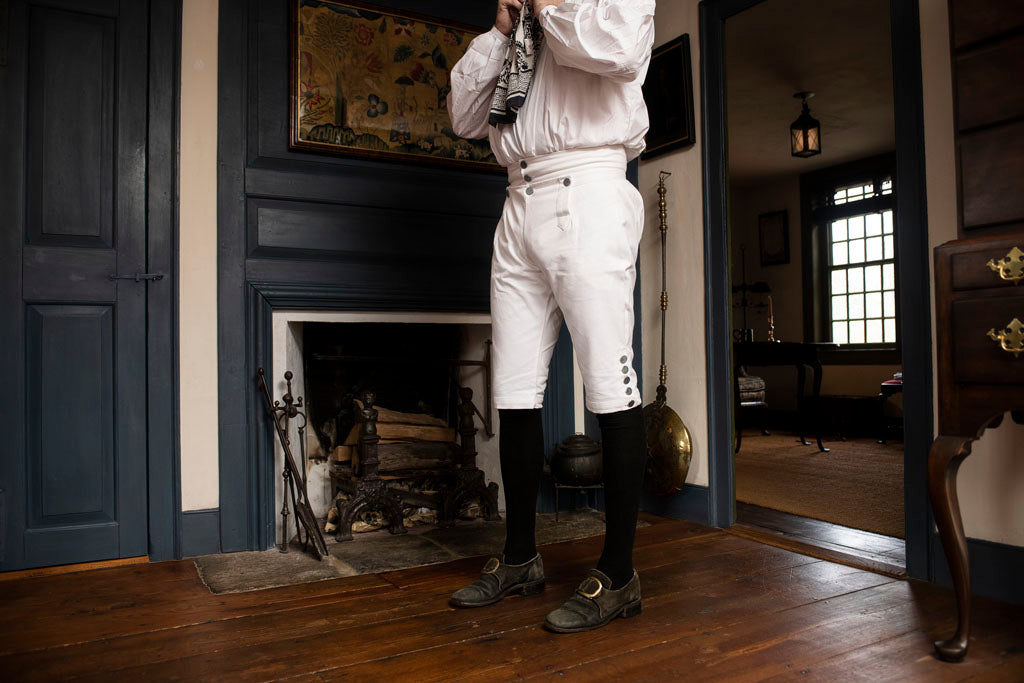A man, dressed in an old-fashioned jockey or colonial-style costume, stands prominently in the center of a room, positioned in front of a fireplace. He is clad in a white outfit that includes knee-high black socks and brown leather shoes featuring large gold buckles. His white shorts are intricately detailed with buttons at the waist and leg seams, tightly fastened. He wears a tucked-in white shirt and appears to be adjusting a black and white scarf around his neck, though his face is not visible.

The room's interior is detailed and vintage. To the far west, there's a bluish-black door with a white strip beside a fireplace painted in the same hue. Positioned above the fireplace is a dominant yellow-shaded painting with a unique design. The inside of the fireplace is white, holding stacked pieces of brown wood. Gray stone pieces are embedded into the multi-shaded brown floor in front of the fireplace. 

Behind the man, an open door leads into another room illuminated by natural light from a window and a brown ceiling light fixture. This adjacent room has a dark tan carpet, with a table on its left side. Back in the main room, to the left of the fireplace, you can partially see a dresser with golden handles on the bottom two drawers. This meticulously detailed image not only captures the man's anachronistic attire but also the antique and thoughtfully decorated setting that surrounds him.